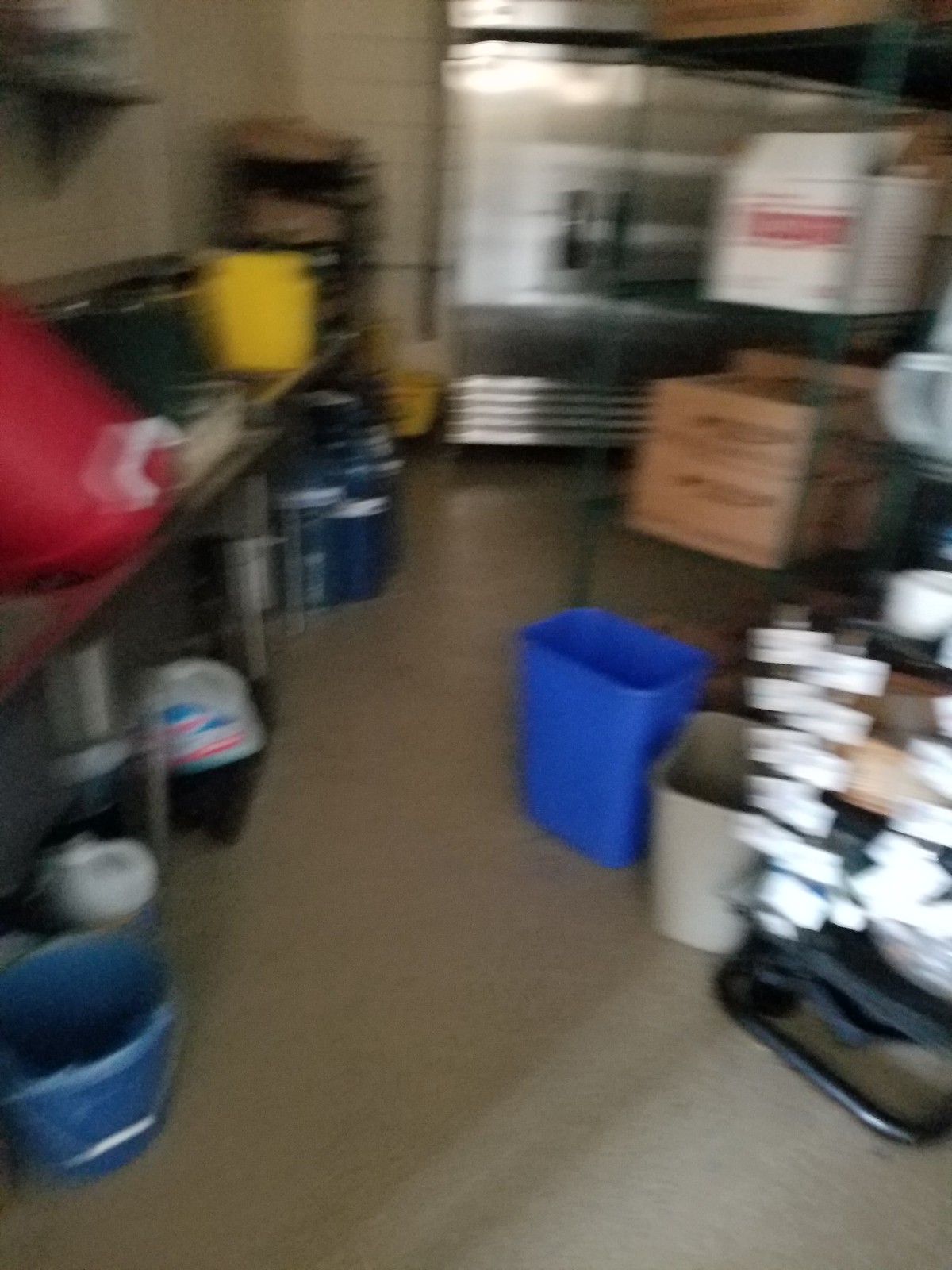The image depicts a somewhat blurry view of a room that appears to be a storage area or part of a kitchen. The floor is tiled in a light beige color. Dominating the background, there's a large chrome refrigerator with three or four doors, accompanied by a rack that may be storing bread. On the left side of the room, there's a set of storage shelves piled up with some boxes, including a white one on top of a brown one. Nearby, there are small blue and beige trash bins made of plastic or resin. Further details include a stone brick wall, a counter with several buckets—highlighting a red and a yellow one—and a hard hat possibly situated under the counter. There is also a blue mop bucket on the floor, potentially some bleach underneath sinks along the side, and some additional small blue and gray trash bins. On the top shelf, a larger red item and another yellow bucket can be observed.